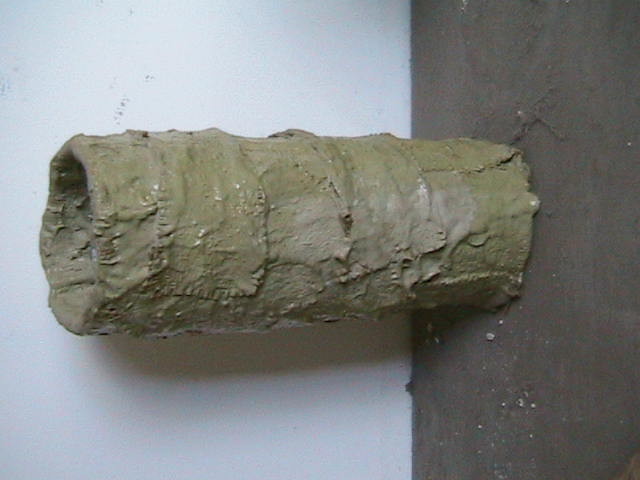The image depicts a cylindrical object resembling an empty toilet paper roll or pipe, covered in a mix of khaki, green, and gray, giving it a dirty, irregular appearance. The cylinder, which may be wrapped in fabric or paper and possibly painted, extends from a dark brown or gray surface and protrudes over a white or very light blue wall, suggesting an indoor setting. The open end of the hollow cylinder hints at a function like that of a drainage pipe or dryer attachment, though its exact purpose remains unclear. The ground beneath is brown, adding to the overall earthy, muddy aesthetic.